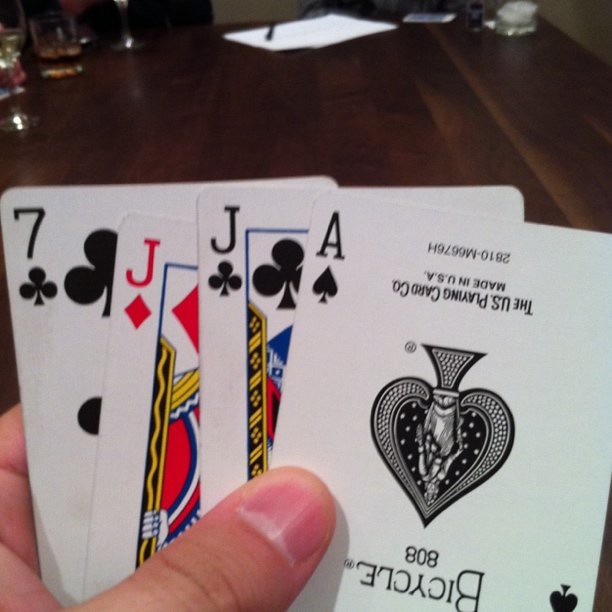A square color photograph captures a close-up of a hand holding a set of playing cards. Emerging from the lower left corner, the hand features light skin and very short fingernails, which are slightly flushed pink. The visible index finger is shown from the bottom, while only the top of the thumb is seen. The hand grips four cards, delicately fanned out horizontally: the seven of clubs, jack of diamonds, jack of clubs, and the ace of spades. 

In the upper portion of the image, a dark brown wooden table, with its grain panels subtly angled leftward, serves as the backdrop. Towards the top edge of the table, a white piece of paper lies, slightly askew to the right, with a black pen placed atop it. Two clear drinking glasses filled with a golden liquid rest on the upper left side, while a silver object, possibly a coaster, is situated on the upper right.